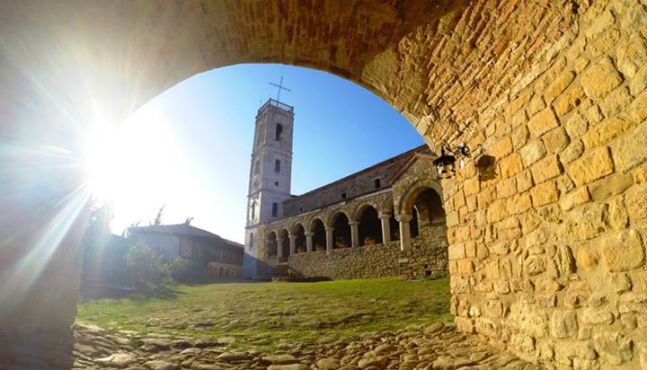This landscape-oriented color photograph captures the view from inside a stone tunnel looking out towards an ancient church. The tunnel, constructed from beige hand-cut stones, features a large arched opening with a stone floor. A lamp post is mounted on the right side of the tunnel's wall. Sunlight streams through the top left corner of the archway, creating radiating beams of light accentuated by a star filter effect which bathes the scene in a golden glow on the right-hand side while leaving the other side in shadow.

Outside the tunnel, a grassy area stretches towards the horizon where the church building stands prominently on the right. This church has numerous archways and features a four-story rectangular tower with a cross atop. Attached to this structure are more arched columns under a shorter section. Another building is visible to the left of the steeple. The sky through the archway is a clear blue, enhancing the scene’s serene and timeless atmosphere.